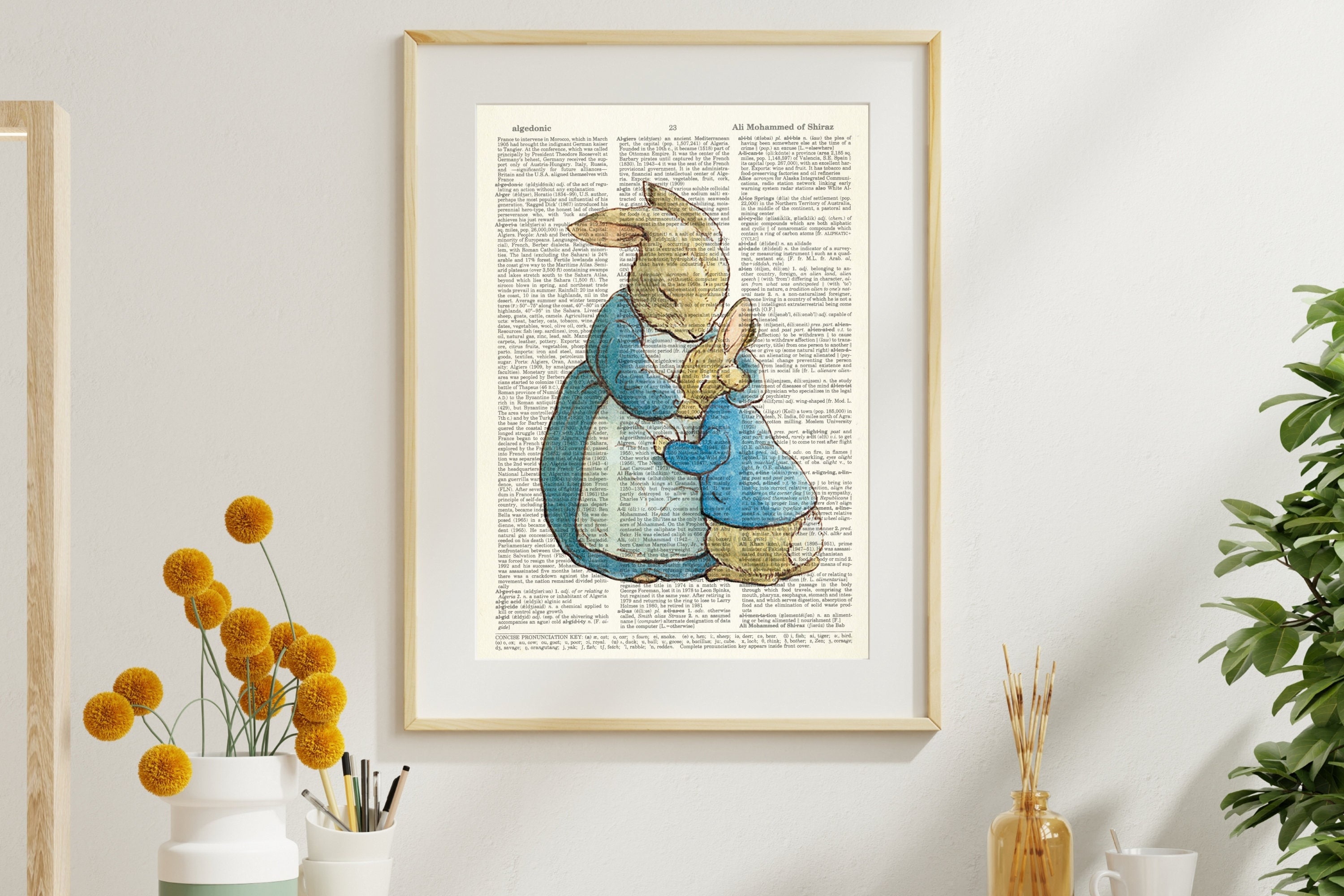The image depicts an interior scene with an off-white, grayish-white wall as the backdrop. Centered on the wall is a framed picture with a thin, light tan-colored frame, showcasing a page from a children's book. The text on the page is unreadable, but prominently featured is a transparent illustration of an adult bunny embracing a baby bunny. The mother bunny, with closed eyes and ears laid back, wears a red dress and a whitish apron, while the baby bunny, face nestled into the mother's chest, is clad in a blue jacket, revealing a small white bunny tail.

Below the picture, a countertop is partially visible, adorned with various objects. To the left, a white vase holds vibrant orange, pom-pom-like blooms with green stems, and nearby, a pencil holder brims with an assortment of pencils. To the right of the picture, a diffuser with several sticks protrudes from a jar, standing next to a white coffee cup. Flanking the far right edge of the frame, vertical green plant leaves, likely from a fake plant, subtly intrude into the scene.